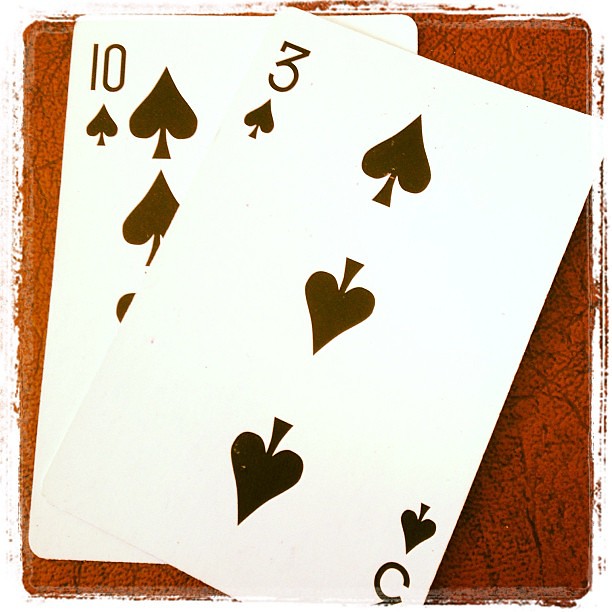This image features an artistic depiction of two playing cards—the 10 of Spades and the 3 of Spades—arranged in a layered composition. Both cards are shown in black and white, with the spade symbols and numerical values rendered in a bold black against a stark white backdrop. The 3 of Spades lies diagonally across the 10 of Spades, creating an overlapping effect that adds depth to the composition. 

These cards are set against a textured brown background that resembles a wooden table, complete with black streaks to enhance the effect. The cards themselves are outlined with a white border, subtly tinged with brown to blend seamlessly into the background.

The image appears to be digitally created, with a polished and clean finish, making it an ideal candidate for various formats such as prints, posters, or even metal signs. The attention to detail in this artwork suggests it is designed for visual appeal and decorative purposes.